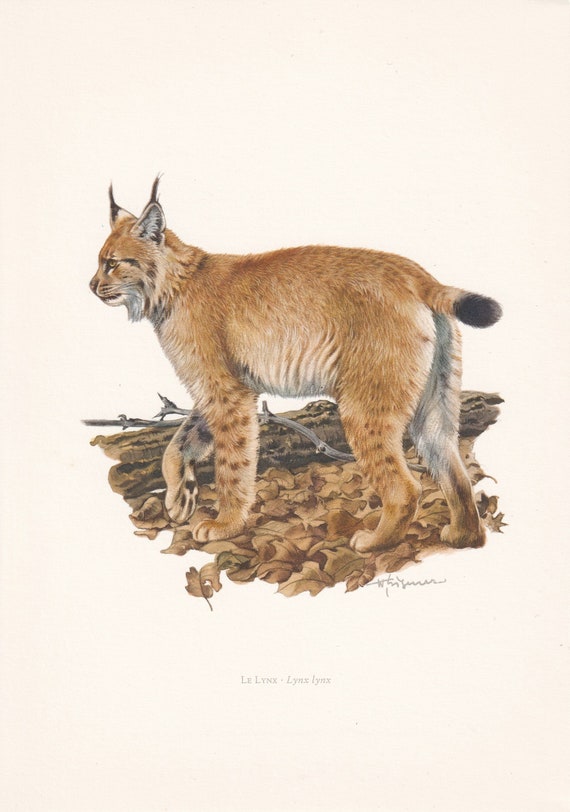This artwork depicts a detailed, colored image of a lynx cat. The lynx, captured in a naturalistic style suggesting either painted or colored pencil techniques, features orange fur with a white underbelly and hind parts. Its legs showcase black and white spots, with some spots appearing more like dots or stripes. The lynx has distinctive black-tipped ears and a short tail that also ends in a black tip. The animal is depicted standing amidst a bed of tan-colored leaves, in a scene that includes a fallen tree trunk and some branches on the ground, suggesting a woodland environment. The lynx’s gaze is directed to the left, and it has one front paw raised, poised as if ready to walk forward. The background is a solid beige color. Below the image, the text "Lynx lynx" is visible, which appears to be either a title or an autograph from the artist.